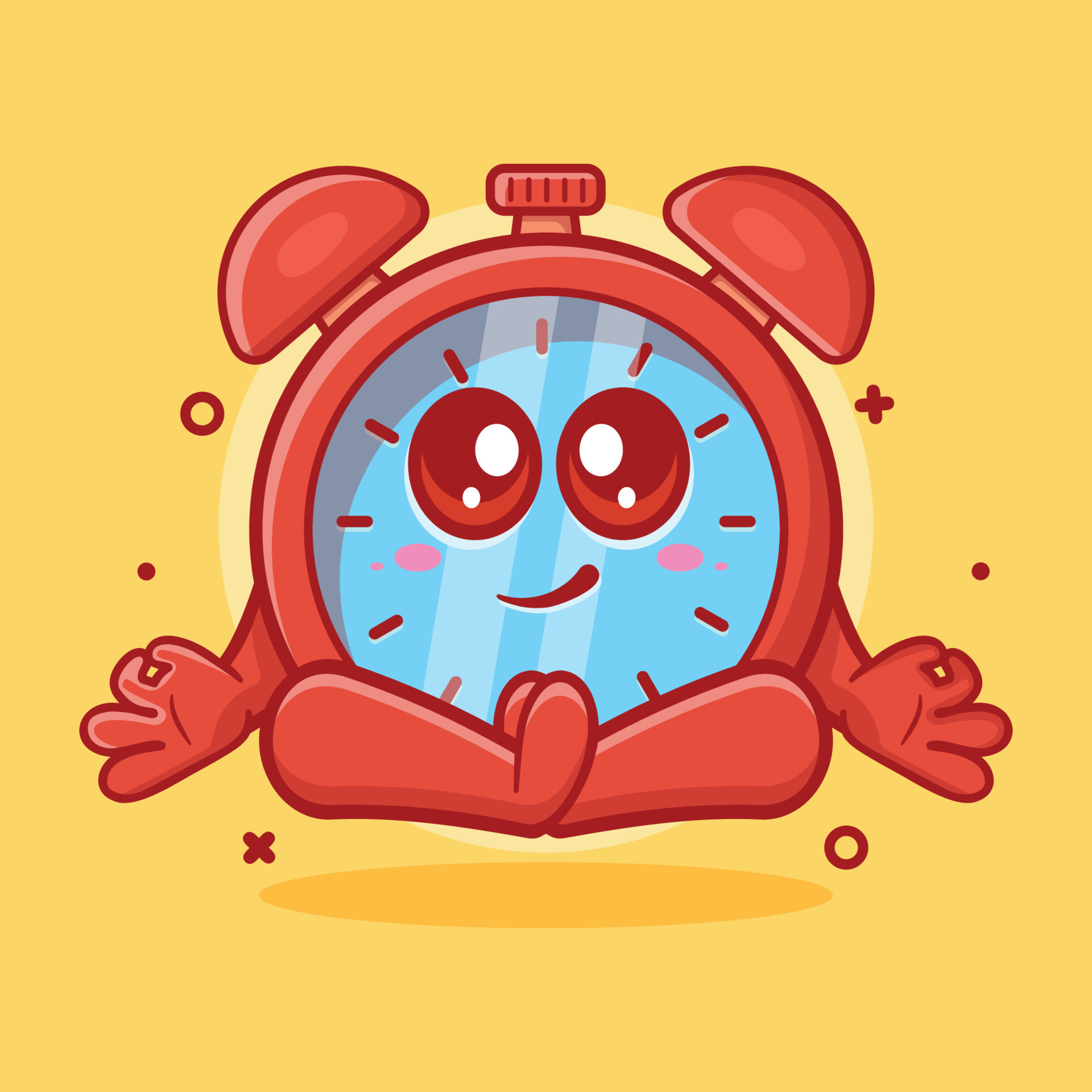This image is a cartoon-style graphic featuring a red alarm clock sitting in a lotus position against a bright yellow background. The clock, stylized with gradient shades from dark orange to red, has a face adorned with pale blue stripes transitioning to lighter blue. It appears content, displaying a slight smile and white eyes with pink patches on its cheeks. The clock is depicted with anthropomorphic features, including hands and legs locked in the meditative lotus stance, with its fingers forming the 'okay' gesture. Surrounding the cheerful clock are various symbols: an X and an O at the bottom and an opposite X and O near the top near the alarm bells. A lighter yellow circle behind the clock adds a sense of depth, and a subtle shadow beneath it enhances the three-dimensional effect. Overall, the vivid and animated design conveys a serene, happy demeanor.